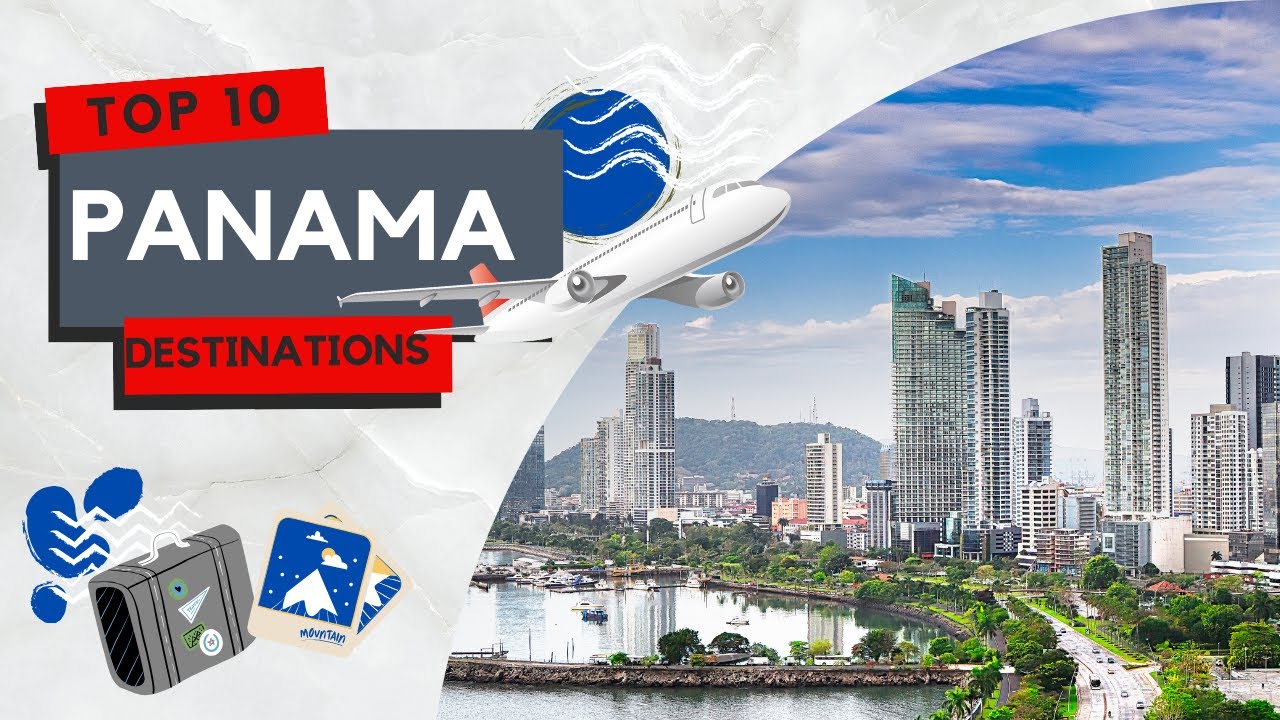The image is divided into two distinct sections, blending artistry and travel elements in a captivating manner. On the left, a cartoonish, non-animated background sets a playful tone with curved lines creating a distinctive, diagonal separation. The right-hand side prominently features a bustling cityscape, depicting a large urban area teeming with skyscrapers and notable landmarks. The scene showcases a vibrant waterfront, dotted with numerous boats and jetties extending into the water, highlighted by a highway running along the waterfront’s edge. A majestic mountain forms the backdrop, standing tall under typical fair weather skies filled with blue hues and scattered clouds. 

Complementing this picturesque view, the left side presents a collage of travel-themed text and visuals. The bold title "Top Ten" is set against a vivid red background, followed by the name of the country "Panama" on a more understated gray backdrop. The word "Destinations" appears again on a red background, emphasizing the theme. Adding to the travel motif, stylized graphics such as an airplane, a postmarked stamp, postcards, and a suitcase are interspersed, evoking a sense of adventure and exploration.